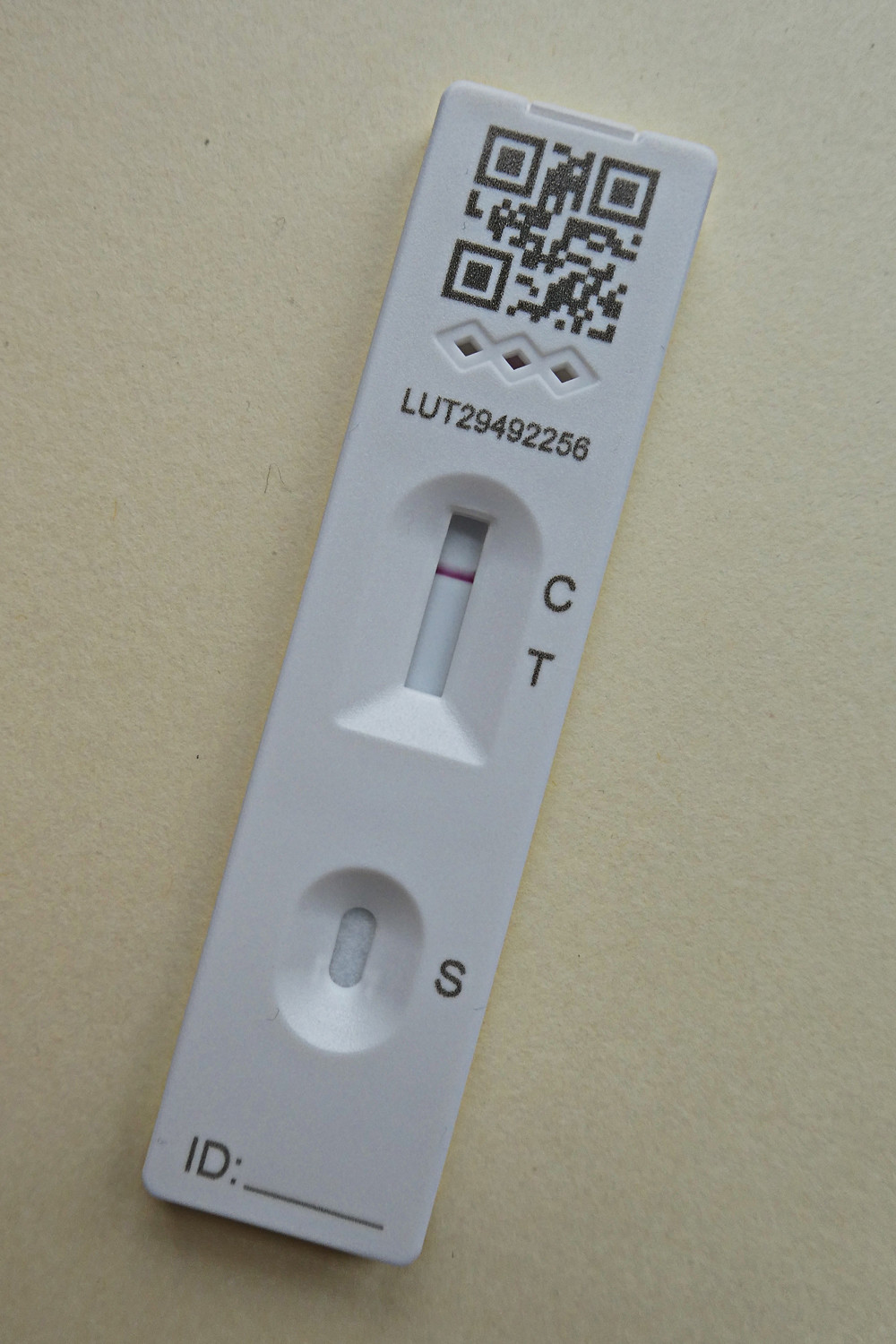The image depicts a white pregnancy test, positioned diagonally from the top right to the bottom left against a white background. The test is predominantly white with a centered slit near the top. Just below this slit is a small square QR code, which contains two black squares in the top left and top right corners, another in the bottom right corner, and three smaller diamond-shaped cuts within the code. Underneath the QR code, the alphanumeric sequence "LUT29492256" is printed in black text.

Below this text, there is a rectangular display area with a red line running horizontally across it at about two-thirds up from the bottom. To the right of this red line is the letter "C" and below it is the letter "T." Further down, the test has a rounded rectangular section, which is blank inside, and to its right is the letter "S." At the bottom of the test, there is an "ID:" label followed by a blank line meant for writing a name or initials.